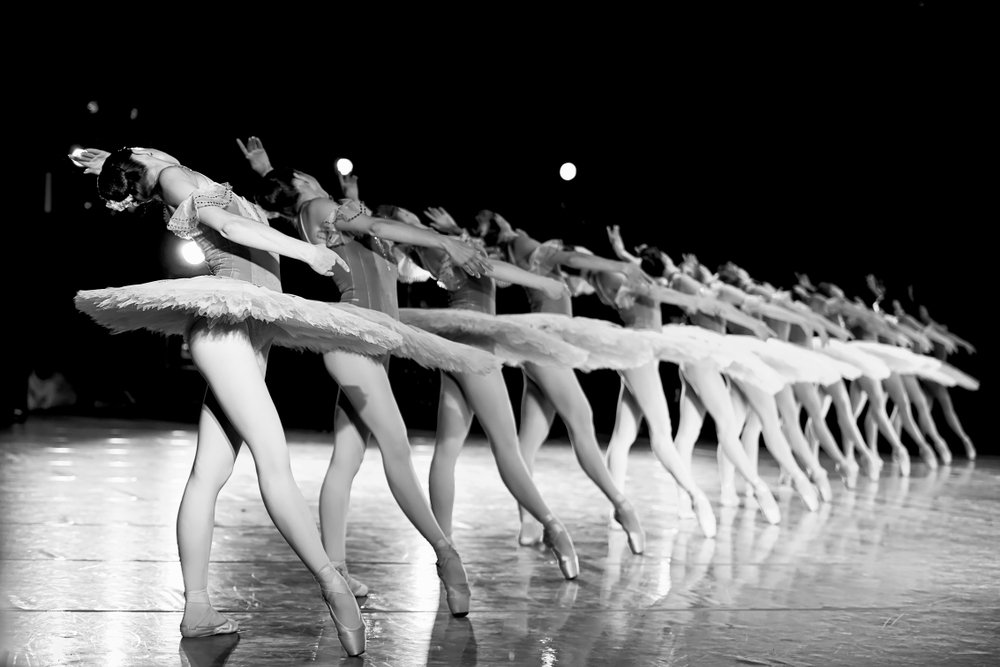In this black-and-white photograph, a line of approximately 20 ballerinas elegantly holds a synchronized pose against a shiny stage. The dancers, all women with dark, up-styled hair, are clad in identical costumes consisting of grey leotards and wide, fluffy skirts that fan out dramatically, almost horizontal. They stand in a diagonal formation, beginning from the bottom left corner and extending towards the right, about a quarter up the image. Each ballerina has her left leg extended in front on tiptoe while the right leg is positioned back and to the side, flat on the floor. Their right arms are extended backwards with their heads and torsos gracefully tilted backwards. The stage is enveloped in darkness with a bright, circular spotlight illuminating the scene from above the dancers' heads, enhancing the composition of this striking visual.